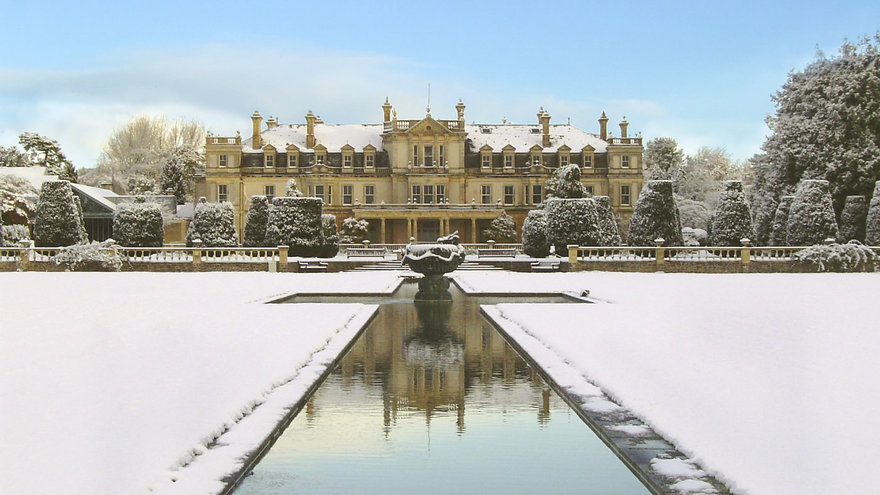The image showcases a grand, old-style mansion, constructed from light yellowish-brown stone and accentuated with tan and brown detailing. This three-story mansion features a slanted roof piled with freshly fallen snow, rectangular windows on the second level, and arched windows on the third level, which protrude slightly from the main structure. Below the mansion, there's an inviting flat-roofed entrance supported by columns.

In the foreground, a stately cross-shaped pond stretches out towards the mansion, spanning roughly 50 feet. At the intersection of the cross stands a prominent fountain, its design reminiscent of a grand, thick wine glass. The water in the pond is a dark, muted grayish-brown, adding a reflective quality to the scene. The fountain, although currently not operating, directs attention towards the mansion's elegant stairway leading into the house.

The photograph, taken during the daytime, captures the winter season in full effect. Snow covers the ground, the rooftop of the mansion, and the meticulously trimmed hedges, which resemble trees with flat tops. Adjacent to the courtyard and surrounding the mansion are several bare, flat-topped trees, all blanketed in smooth, untouched snow. The sky above is a pale blue, dotted with low-lying grayish clouds, adding a serene and crisp atmosphere to this picturesque winter scene.